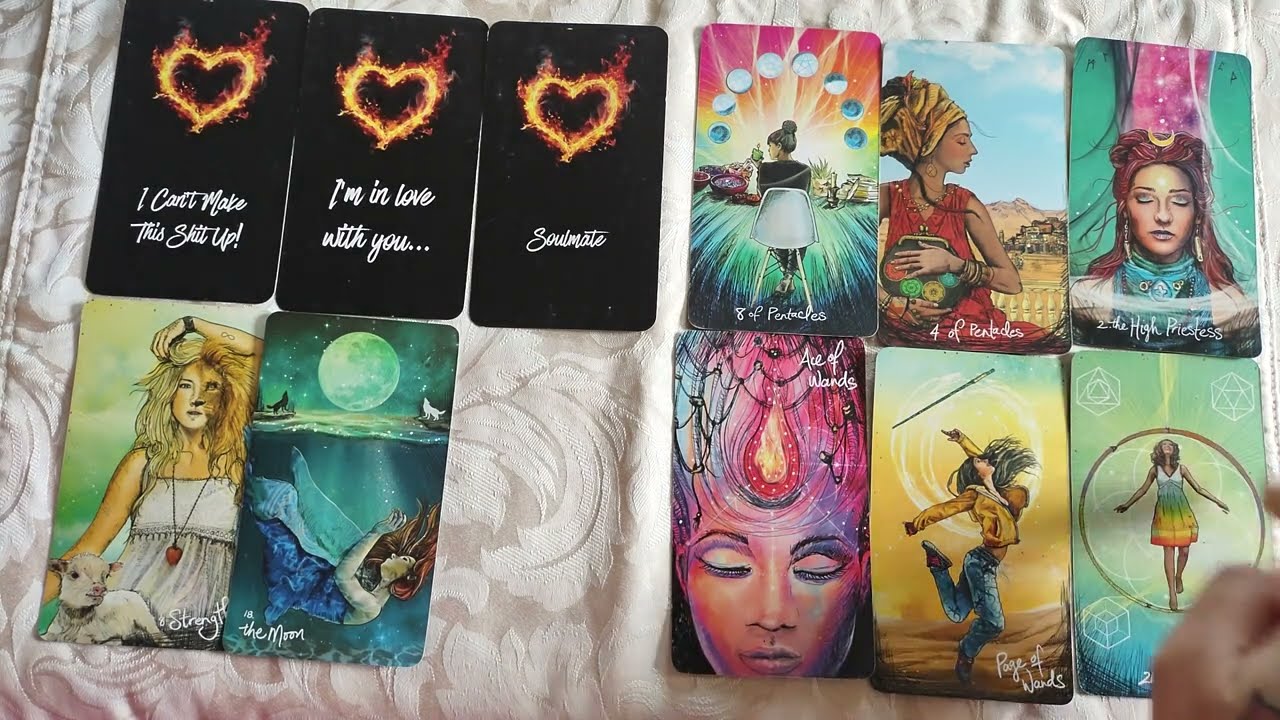This image is a colorful, detailed photograph of 11 vertical rectangular cards with rounded edges, laid out horizontally on a fabric with a white and silver floral design. In the bottom right corner, a blurred person's hand can be seen. The cards appear to be a mix of affirmation or tarot-inspired cards featuring vibrant illustrations and geometric designs.

On the top row, the first three cards are black with a heart shape surrounded by flames at the top and white text at the bottom. The texts read, from left to right: "I can't make this shit up," "I'm in love with you," and "Soulmate." To their right, there are three more cards: one depicts a woman seated in a chair, the next features a woman with a head wrap holding a bag in a desert setting, and the third shows a woman with her eyes closed, adorned with a moon on her forehead and stars above her head.

The bottom row has five more cards. The first card on the left illustrates a woman with blonde hair holding a lamb, partially transforming into a lion. Next to it is a card with a woman submerged underwater with a moon above. The middle card showcases a woman with a large pink jewel on her forehead. Following that is an illustration of a woman dancing with her long hair flowing upwards. The final card on the right depicts a woman inside a circular frame surrounded by geometric shapes.

The various styles and themes of these cards, combined with their placement on a floral fabric, create a visually engaging and eclectic scene.